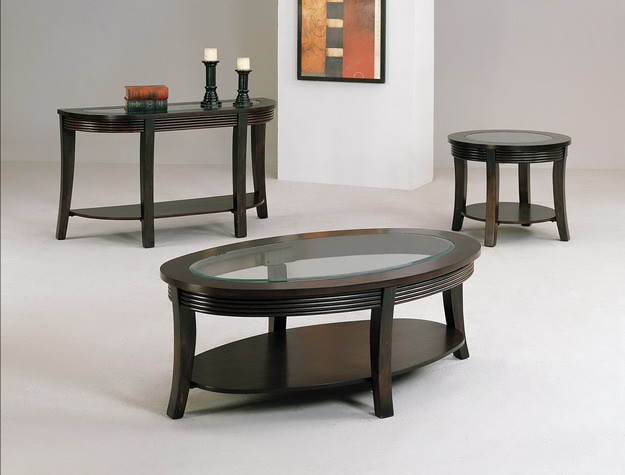This professionally-shot photograph, likely intended for a furniture company or interior design catalog, showcases a set of matching dark wood tables in a meticulously lit studio room with white walls, casting minimal shadows. The central focus is a vertical, flat white pillar displaying a piece of framed abstract art. The art features a black frame enclosing textured shapes: a burnt orange rectangle on the left, a brick red one on the right, and thick black stripes almost covering an ivory rectangle in the middle, all bordered by thin white lines.

In the foreground, there's an oval coffee table with a glass top and a lower shelf just above the floor. It features intricate fluting along the edges and stands on four legs. To the left, a demi-lune shaped hallway table or sideboard carries two dark wood candlesticks with white pillar candles and a decorative statue resembling a stack of books. This table also has fluting along its edge and a lower shelf.

To the right, there's a matching round side table with a glass inset top and a lower shelf, maintaining the same dark wood, four-legged design, styled in harmony with the other pieces. The cohesive design and rich dark cherry finish of the furniture pieces are complemented by the art, emphasizing the sophisticated yet inviting aesthetic of this showroom or catalog setup.